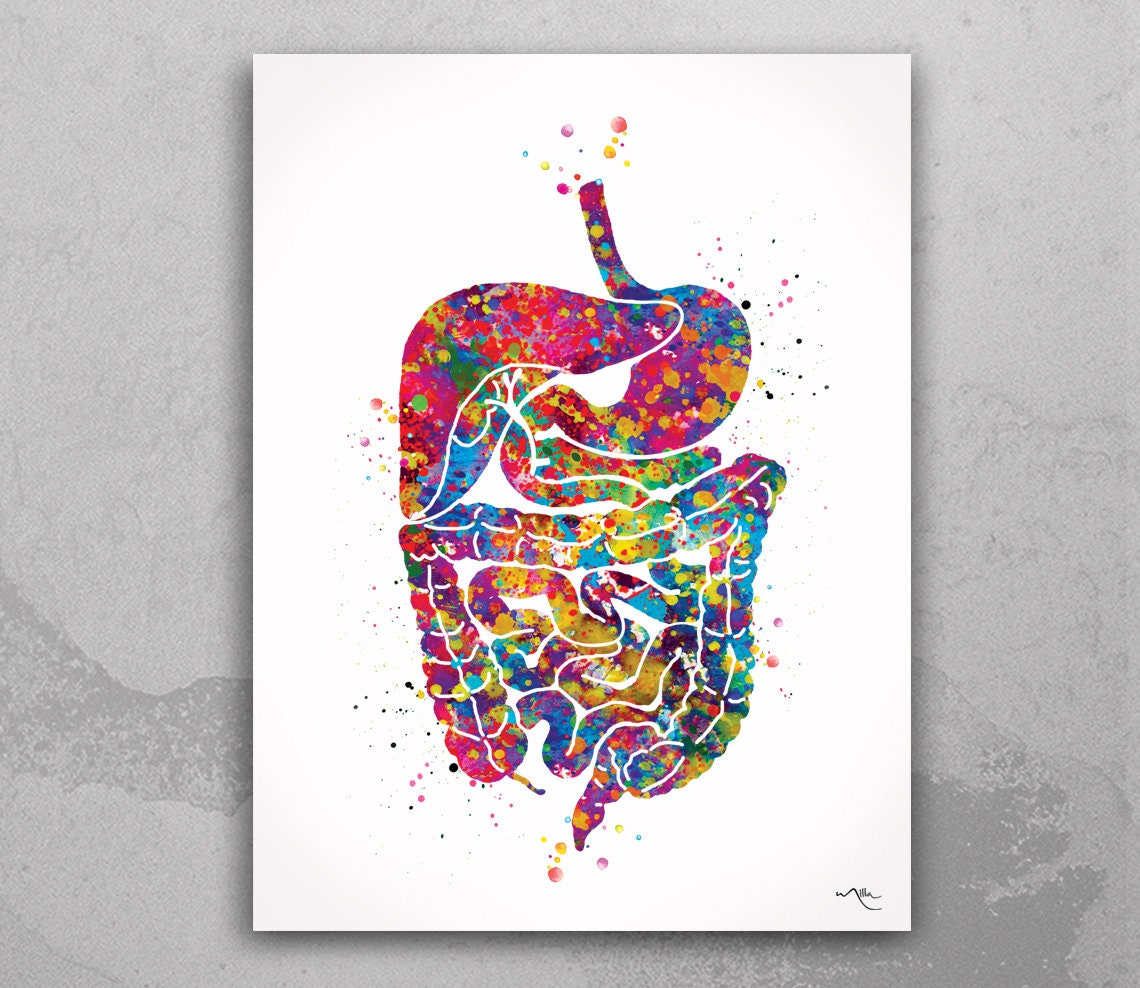This painting vividly illustrates the human digestive system with a whimsical, abstract twist. Set against a totally white canvas, the artwork depicts key digestive organs, including the stomach, liver, and intestines, all rendered in a vibrant, Jackson Pollock-inspired style. Splashes of color—red, orange, yellow, green, blue, purple, magenta, and teal—decorate the entire digestive tract, from the esophagus (cut off at the top with dots of color emanating) to the large intestine (with similar color dots at the bottom). The artist's chaotic splotching bridges the various parts, blending them into a cohesive yet abstract representation. The canvas, rectangular with a gray, imperfectly smooth background, includes the artist's signature in black ink at the bottom.